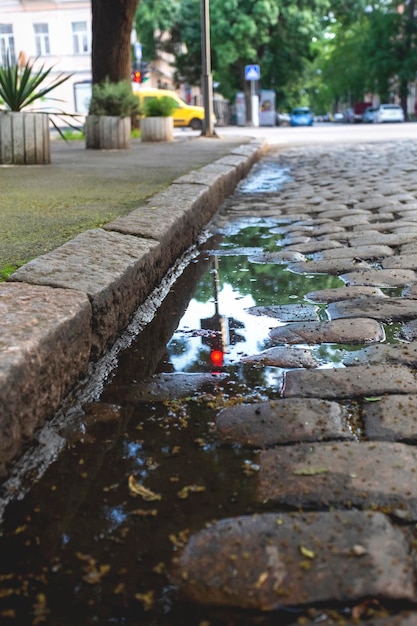The photograph captures a close-up view of a cobblestone street complemented by a curb made of individual granite blocks. A sizable puddle hugs the curb stones on the left-hand side, reflecting the red light of a nearby traffic signal. The scene hints at recent rainfall, evidenced by the water accumulation and raindrop stains scattered across the cobblestones, which are uneven and laden with tree debris and leaves. To the left above the curb lies a sidewalk with several planters brimming with lush green foliage, and a large tree stands behind the second planter. In the background, blurred green trees indicate a verdant setting, while a two-story, yellow stucco building with upper-floor windows can be seen. A yellow cab is parked beside a crosswalk in the upper right corner, facing to the right. Sparse street signs and a blue car facing toward the camera further populate the backdrop, adding subtle urban elements to this tree-lined, tranquil scene.